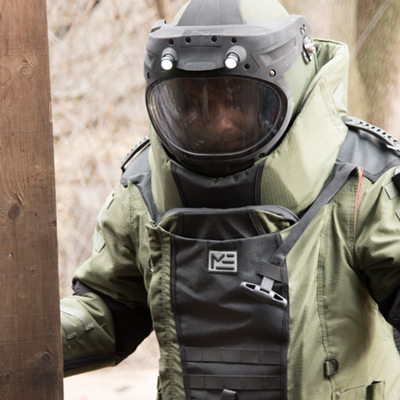In the image, a man stands dressed in a full-body protective suit, reminiscent of hazmat or mining gear. The suit is predominantly olive green with gray accents, and around the shoulders, the green fabric contrasts with gray patches. His outfit features a large, puffy collar that ensures no air penetrates the suit. The helmet, which covers his entire head like an astronaut's headpiece, has a round, reflective glass front that obscures his face, showing only the faint outline of a white man beneath. On top of the helmet are two white circular light sources. The background is a blurred mixture of beige and brown, resembling a dirt wall or hillside, with a vertical wooden plank positioned to the left of the image. His stance is partially obscured, focusing on the upper torso and above, highlighting the suit's robust and encompassing design.